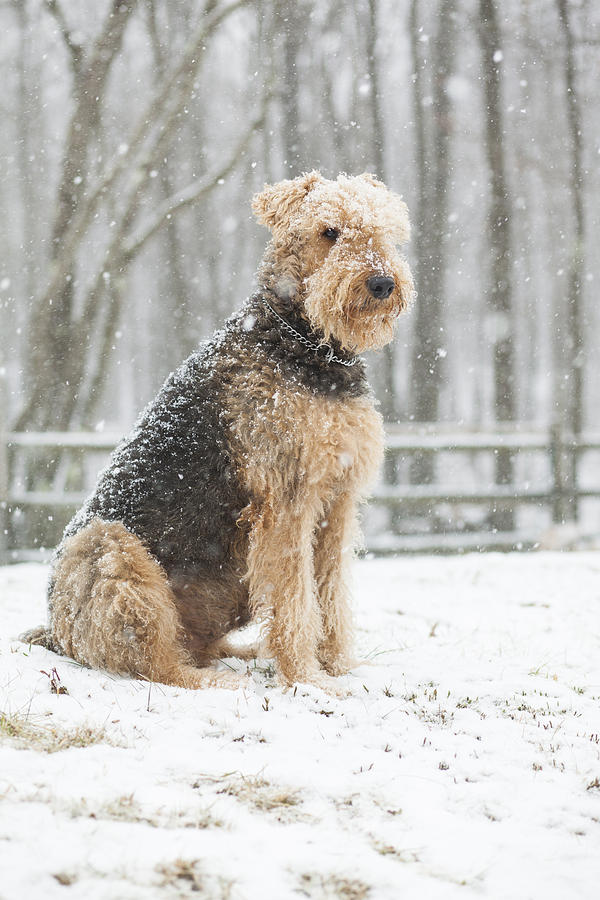The image captures a furry dog, possibly a schnauzer or terrier, positioned slightly left of center and facing right on a snowy day. Snowflakes fall gently around, dusting its light brown fur except for a dark brown, almost black back and neck. The dog, with a single visible eye, subtly turns its head towards the viewer. A silver chain collar adorns its neck. It appears to have been sitting in the snow, which barely covers the ground as patches of dry grass peek through. In the background, a large wooden fence with three horizontal rows of slats stretches across the scene, and behind it, a dense, leafless forest completes the wintry tableau.